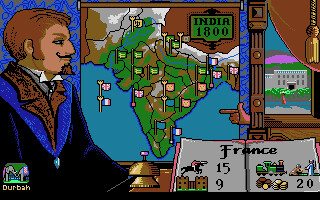This screenshot from a video game encapsulates a detailed historical interface. The small, square image prominently features a Caucasian man with brown hair and a distinctive black handlebar mustache, captured in profile as he gazes to the right. He sports a black jacket highlighted by a blue and red collar. In the bottom left corner, there is a tiny, unreadable icon due to its size.

The man appears to be studying a pixel art map of India, prominently labeled "India 1800" inside a small green square located in the upper right corner. In the lower right section of the image, an open book is perfectly positioned, colored white with "France" spelled out in black font stretching across both pages. The left page of the book displays the numbers “15” and “9”, while the right page presents the number “20”. The pages are accompanied by various small icons, adding to the rich detail of the interface.